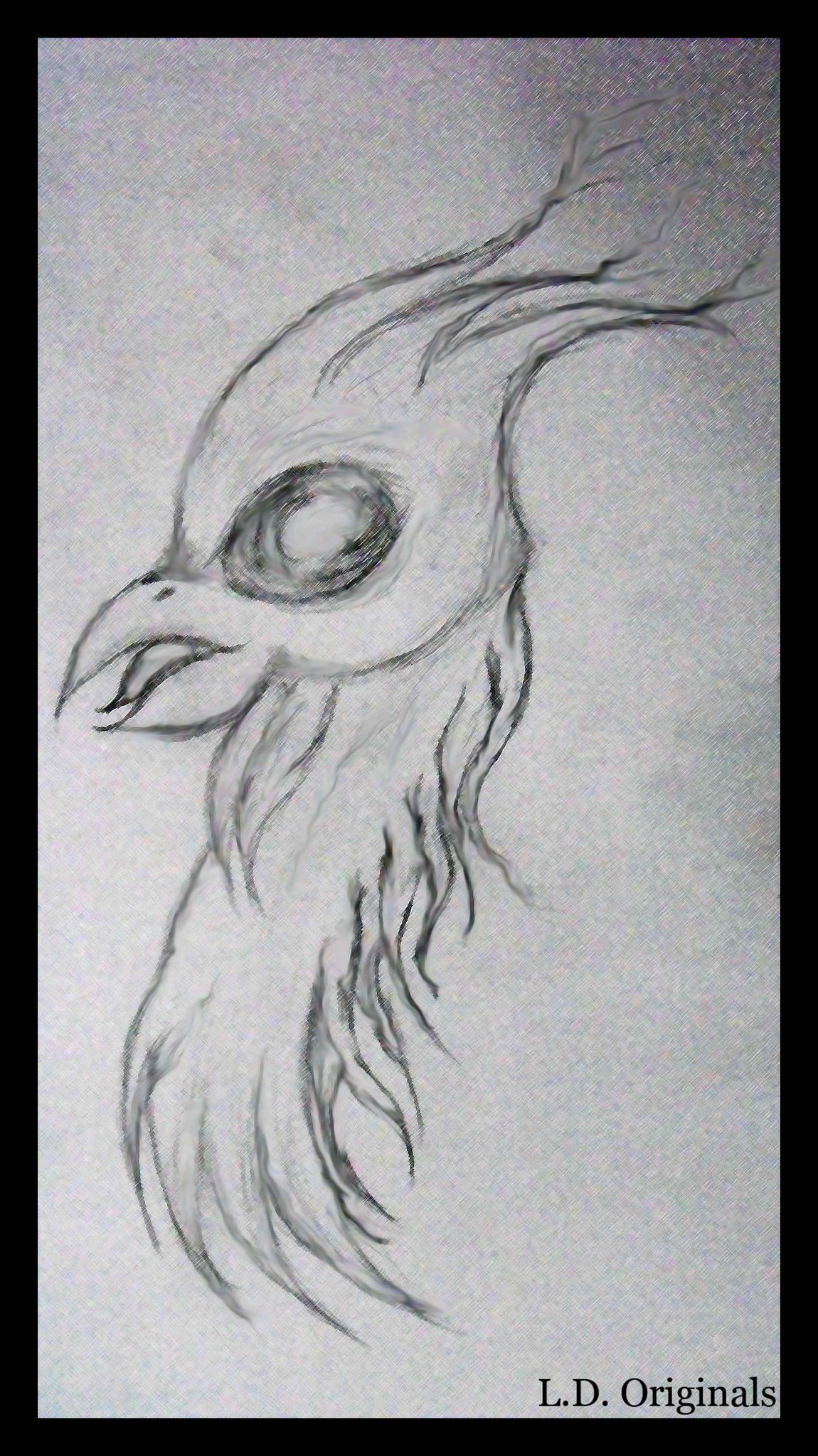The image is a detailed pencil sketch on a white piece of paper that depicts the head and upper chest of a bird, possibly a stylized chicken. The bird's head features an oversized eye with a dark shaded outline and an unshaded white center. Its beak is slightly open, revealing a pointy tongue inside. The top of the bird's head has three peaks of pointy feathers, which extend into flowing, stylized feathers resembling flames. The drawing extends down to show a long, flowing beard-like set of feathers hanging from the bird's neck. The entire sketch has smudged areas, likely from being drawn and handled carelessly. In the bottom right corner, "L. D. Originals" is inscribed, adding a signature to the artwork.